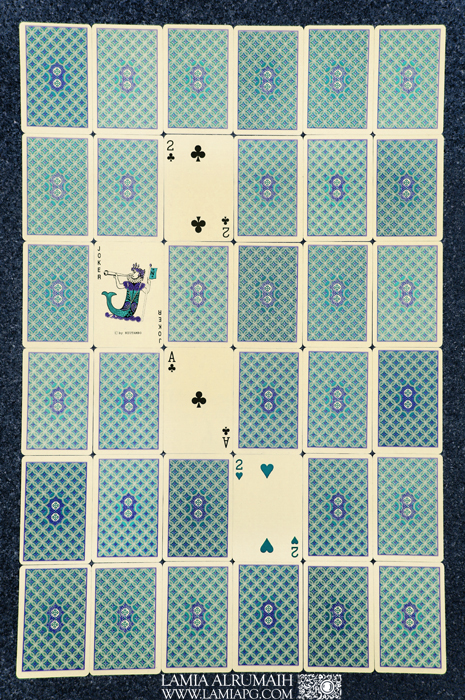In this image, there is a grid of playing cards laid out in a 6x6 arrangement on a dark blue background. The cards are meticulously positioned in rows and columns as follows:

- **Top Row**: All six cards are face down.
- **Second Row**: Two cards are face down, one card (the two of clubs) is face up, followed by three more cards face down.
- **Third Row**: The first card is face down, the second card is a joker card facing up, while the remaining four cards are face down.
- **Fourth Row**: The first two cards are face down, the third card (the ace of clubs) is face up, and the last three cards are face down.
- **Fifth Row**: Three cards are face down, the fourth card (the two of hearts) is face up, displaying a unique blue heart, and the final two cards are face down.
- **Bottom Row**: All six cards are face down.

The backs of the face-down cards feature a distinct blue deck design with intricate blue and white diamond patterns, bordered by a white outline. Additionally, there appears to be a motif resembling two blue circles, one atop the other, which may also be interpreted as an elongated "8" shape.

At the bottom of the image, there is a text in white indicating the name "LAMIA ALRUMAIH." Below the name, a website is listed as "www.lamiapg.com." To the right of this text is a square white spotty rectangle, which appears to be a QR code-like graphic or possibly an abstract design containing a white circle with some rectangular icon inside of it.